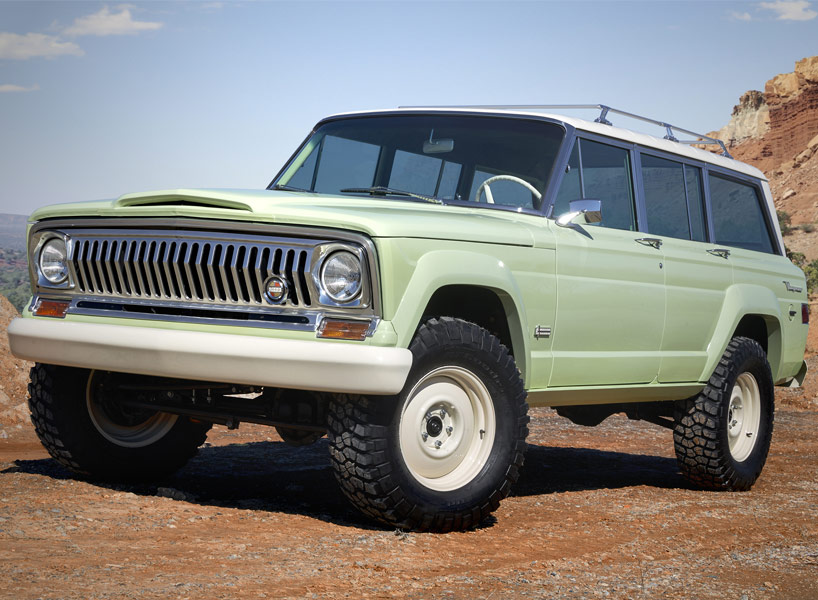This image features a vintage era light green SUV, likely a 1980s model Jeep, perched on top of a hill in a desert scrub environment. The vehicle boasts prominent white accents on its hood, roof, bumpers, and steering wheel, as well as a bright chrome grille with orange turn signals. It rides on four large knobby tires with white rims, emphasizing its robustness for rough terrains. The SUV also sports a silver luggage rack atop its white roof, reinforcing its ruggedness. The background showcases red clay ground and striking red canyon walls under a clear blue sky, enhancing the vehicle's well-preserved and pristine condition in this picturesque setting.